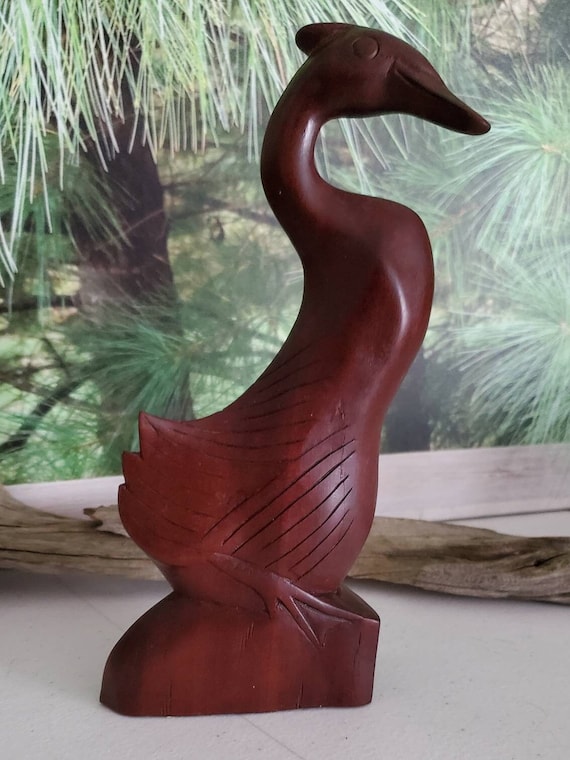The image depicts a finely detailed wooden statue carved in the shape of a bird, most resembling either a crane or a duck, featuring a long neck, elongated beak, and a small crest of feathers on top. The statue is crafted from wood that has a distinguishing reddish hue with carved lines that accentuate the feathering. It is positioned on a beige or white surface, giving it an elegant and simple backdrop. In the background, there's a notable piece of driftwood and a photograph or wallpaper depicting vibrant green pine trees, which contrasts beautifully with the reddish tones of the bird statue. The surrounding details, such as the beige tabletop and the old yet presentable brown table next to it, add depth and context, enhancing the natural ambiance of the scene.